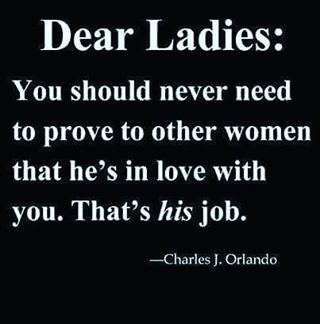On a sleek black background, a light blue quote in elegant mixed-case font reads, "Dear Ladies, You should never need to prove to other women that he is in love with you. That is his job. - Charles J. Orlando." This thought-provoking message, perfect for sharing on social media, setting as a computer lock screen, or integrating with a daily quote app, serves as a gentle reminder to prioritize self-worth and trust in relationships.